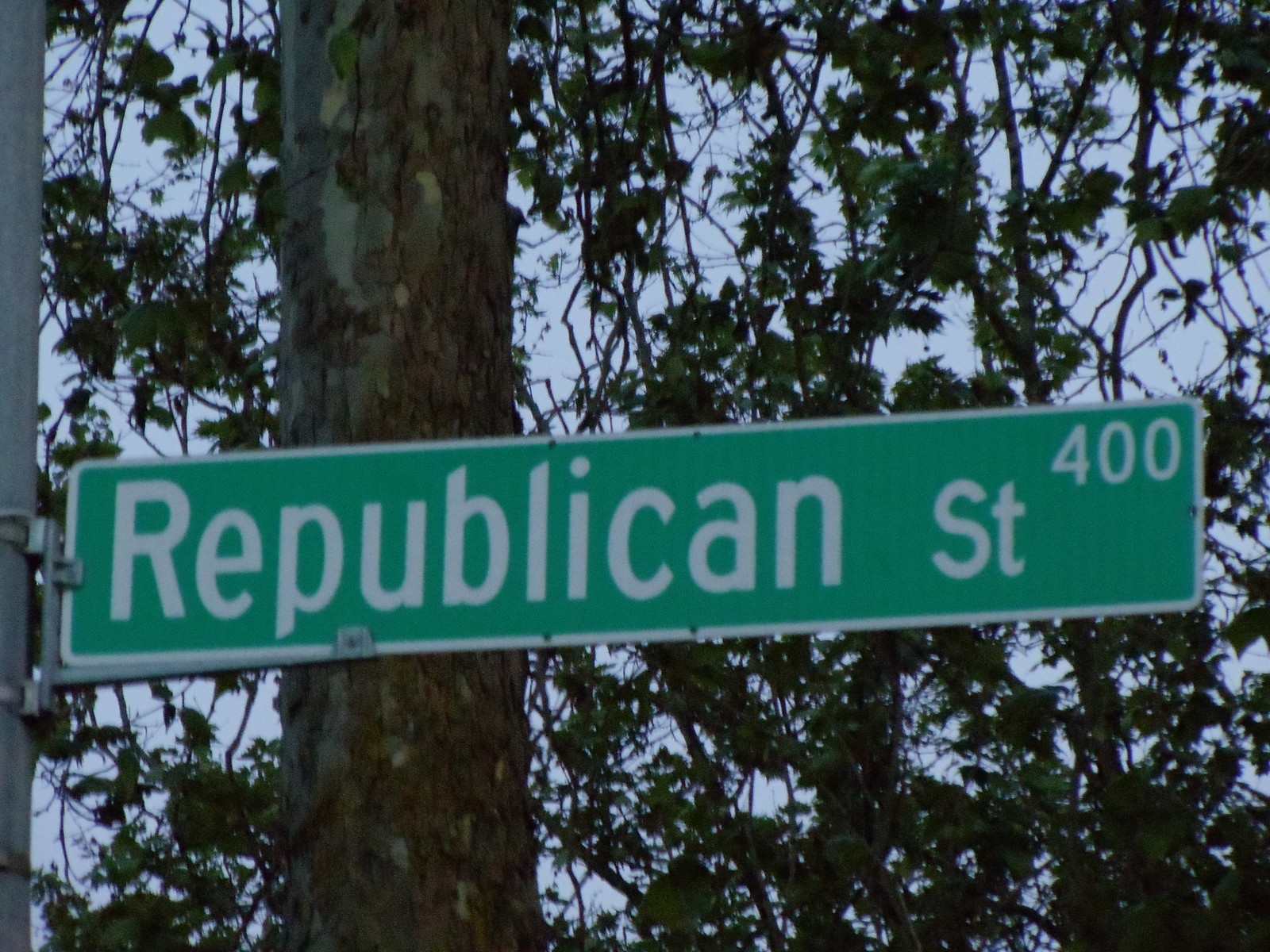This is a detailed, zoomed-in photograph of a street sign. The rectangular sign, which is oriented horizontally, has a green background with white text that reads "Republican Street." In the upper right corner, the number "400" is displayed in white, indicating the block number. A white border outlines the green sign, enhancing its visibility. Although the post is only partially visible, it appears to be made of silver metal.

In the background, there is a brown tree with a skinny trunk. The tree's bark is patchy, with some areas where it is missing, giving it a somewhat bald appearance. The tree's canopy is dense, with numerous branches and an abundance of leaves hanging down.